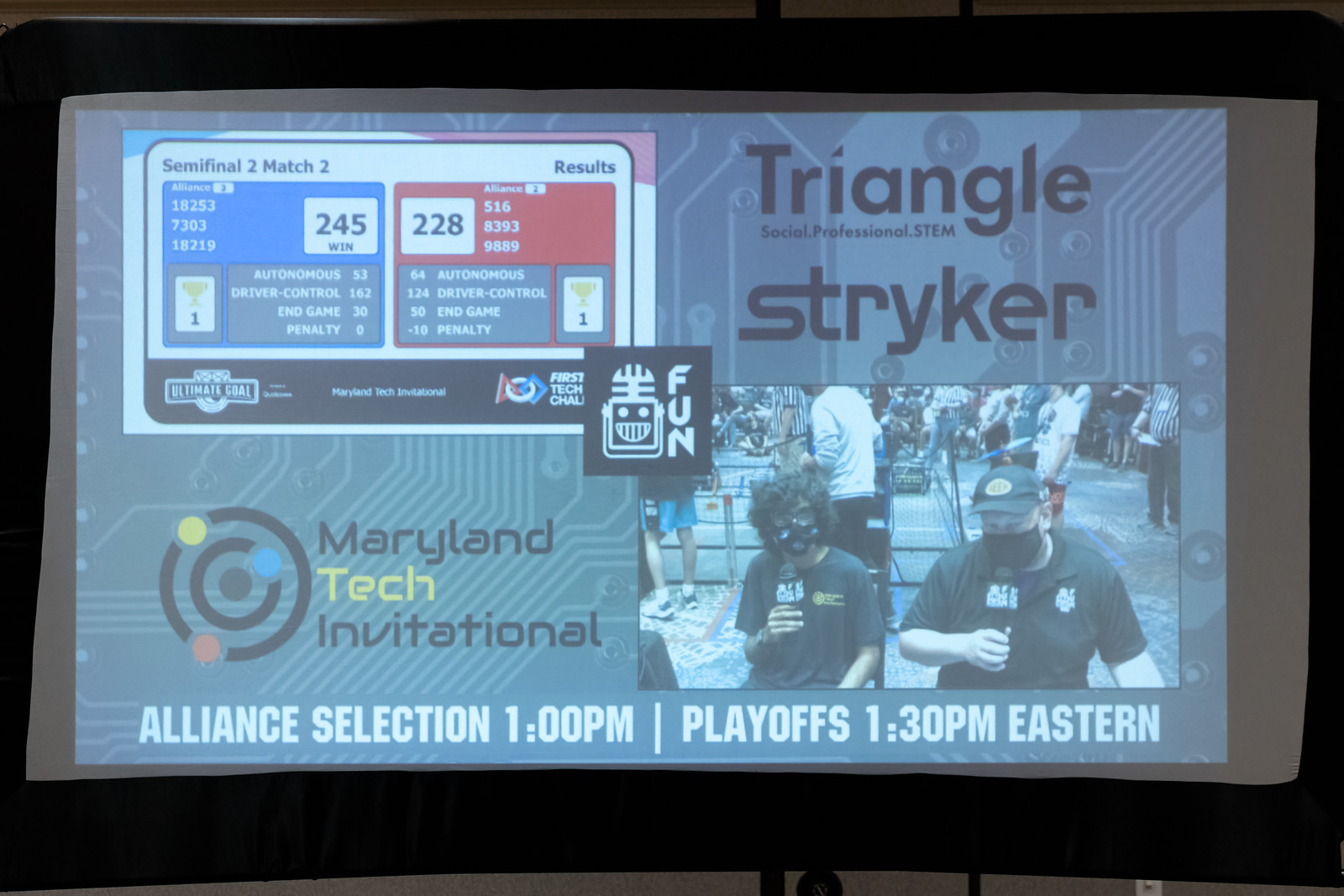The image shows a projected graphic on a screen, likely taken during the Maryland Tech Invitational. The upper left corner displays a scoreboard indicating the results of "Semifinal 2 Match 2." The blue team, with the score "245," marked as the winner, and the red team scored "228." Below the scores, there's a row for penalties on both sides, along with some match statistics. Prominently featured text and logos in the upper right corner include "Triangle" and "Striker," with the phrase "social professional STEM" between them. The bottom section and right side of the graphic mention the schedule: "Alliance Selection 1 p.m." and "Playoffs 1:30 p.m. Eastern." In the bottom right, there's a photograph of two masked men in black t-shirts, one with fluffy black hair and the other wearing a black baseball cap, both holding microphones, possibly participants or announcers at the event. The overall setting appears to be indoors, consistent with a convention or competition, potentially a robotics event.